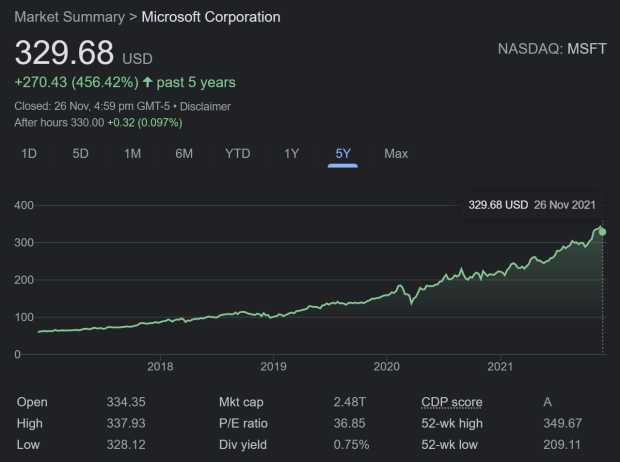This image is a screenshot of a webpage with a dark gray background. The webpage lacks a header or a photograph, making it difficult to identify the exact source. In the upper left corner, the title "Market Summary" is displayed in gray font. Below the title, the text "Microsoft Corporation" appears in white font. Directly beneath that, the stock price for that day is listed as $329.68 USD. Further below, in green, it shows a gain of +$270.43, with a percentage increase of (456.42%) and an upward arrow indicating the movement over the past 5 years.

On the right corner of the screen, the stock exchange symbol "NASDAQ" is visible, along with the stock abbreviation "MSFT". In the center of the screenshot, a graph charts the stock price over a span of several years. The timeline starts on the left with the year 2018, where the price is approximately $100. The graph indicates a significant upward trend, with the price rising to just under $200 by 2020. The stock continued to increase, surpassing $200 in 2021. The graph continues to the right side of the screen, which is marked with the date 26 November 2021, showing the most recent stock price at the end of the period analyzed.